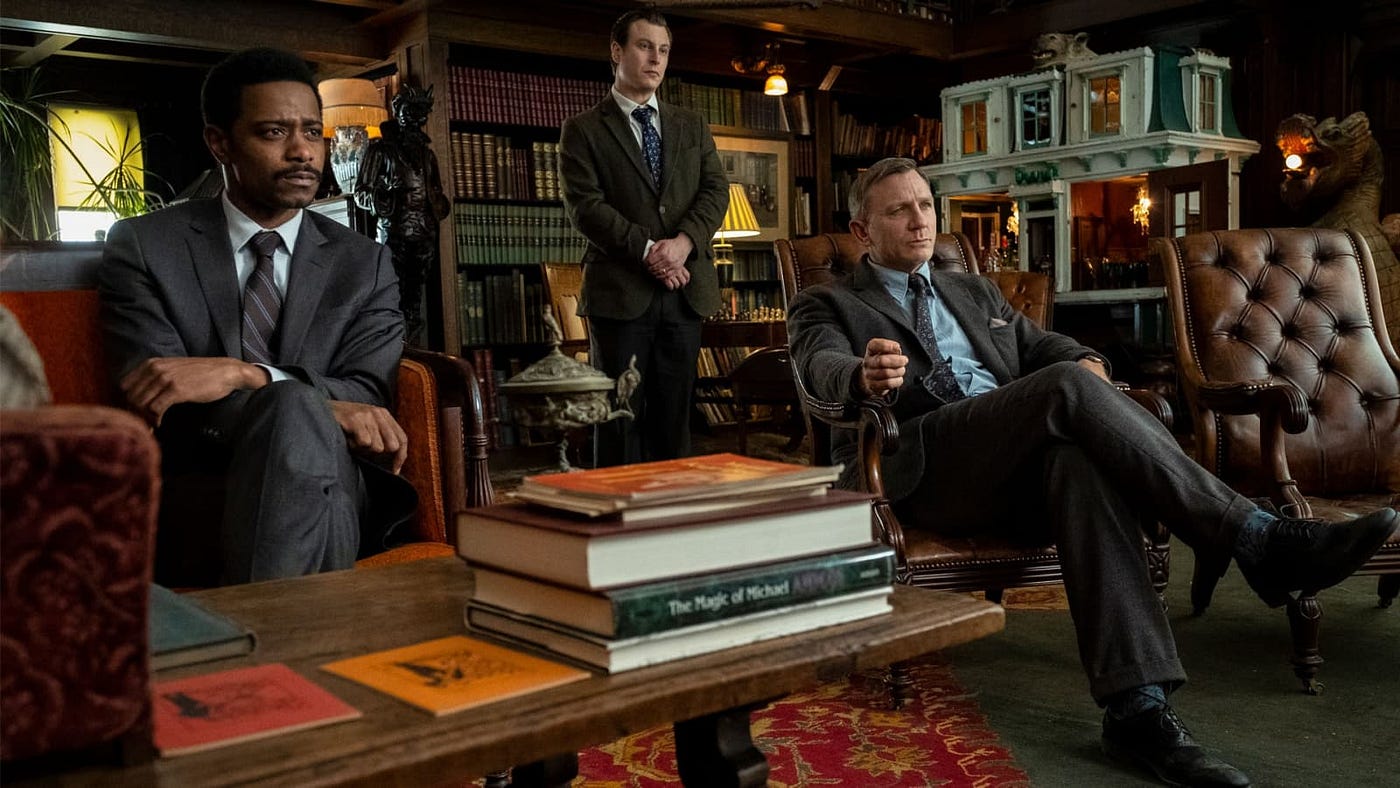The photograph appears to be a scene from a film or TV series, capturing three men in a dimly lit, elegant study or library room. All three men are dressed in suits and display intense expressions as they focus intently on something off-camera. The room features dark wood paneling, statues, and numerous rows of books displayed on a large bookshelf in the background, evoking an atmosphere of sophistication and seriousness.

On the left side, a black man with brown skin, black hair, and a mustache sits in an orange chair, with his arms crossed over his lap and a concerned expression on his face. He is dressed in a gray suit and is seated behind a coffee table stacked with books.

Standing slightly behind him and to his right is a white man in a dark green blazer and dark brown pants. He stands with his arms folded in front of him, in front of the expansive bookshelf.

Seated to the right side of the frame is Daniel Craig, recognizable by his relaxed yet focused demeanor. He sits in a luxurious leather chair, legs crossed, wearing a gray suit paired with a blue shirt and a gray tie. The overall ambiance and decor of the room, combined with the men's serious expressions, suggest an intense or pivotal moment in the narrative.